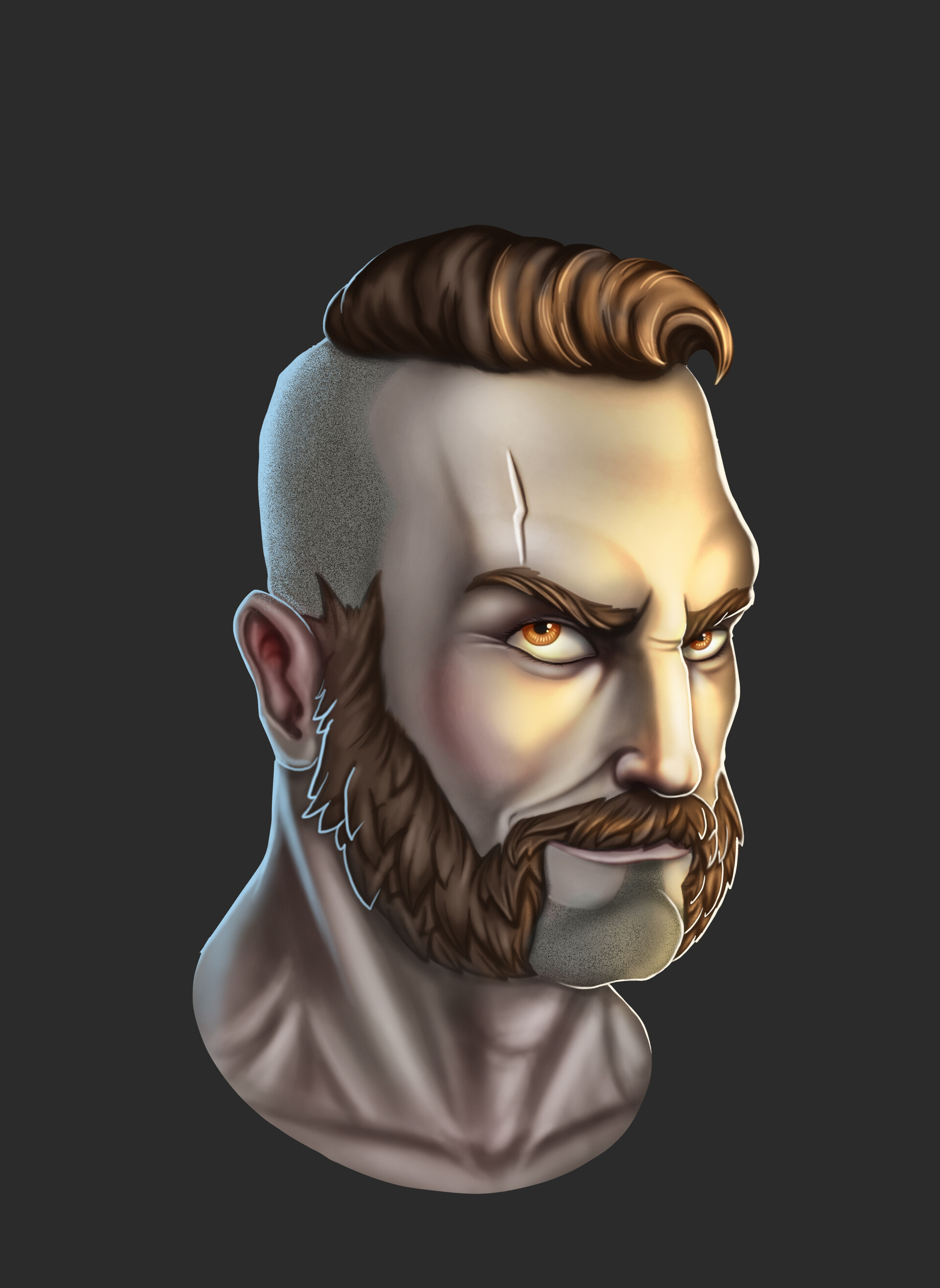This image is a detailed cartoon rendering of a light-skinned man set against a black or grayish background. His hair is brown, styled in a punk fashion with short buzzed sides and a tuft flipped to the right, reminiscent of a mohawk. He has thick brown eyebrows and light, hazel auburn eyes with a furrowed, intense gaze. His face features a prominent, full beard connected to sideburns, which transitions into a handlebar mustache, with the chin shaved to a five o'clock shadow. A distinctive lightning bolt-shaped scar is above his right eye. His neck is prominent and tense, displaying creases. The man's expression is a mix of determination and slight menace, with a subtle smile that suggests he feels ready for a challenge or excited about something. The overall style of the drawing is very shimmery and stylized, with a coppery metallic hue to the skin, emphasizing a non-realistic, graphic art feel.